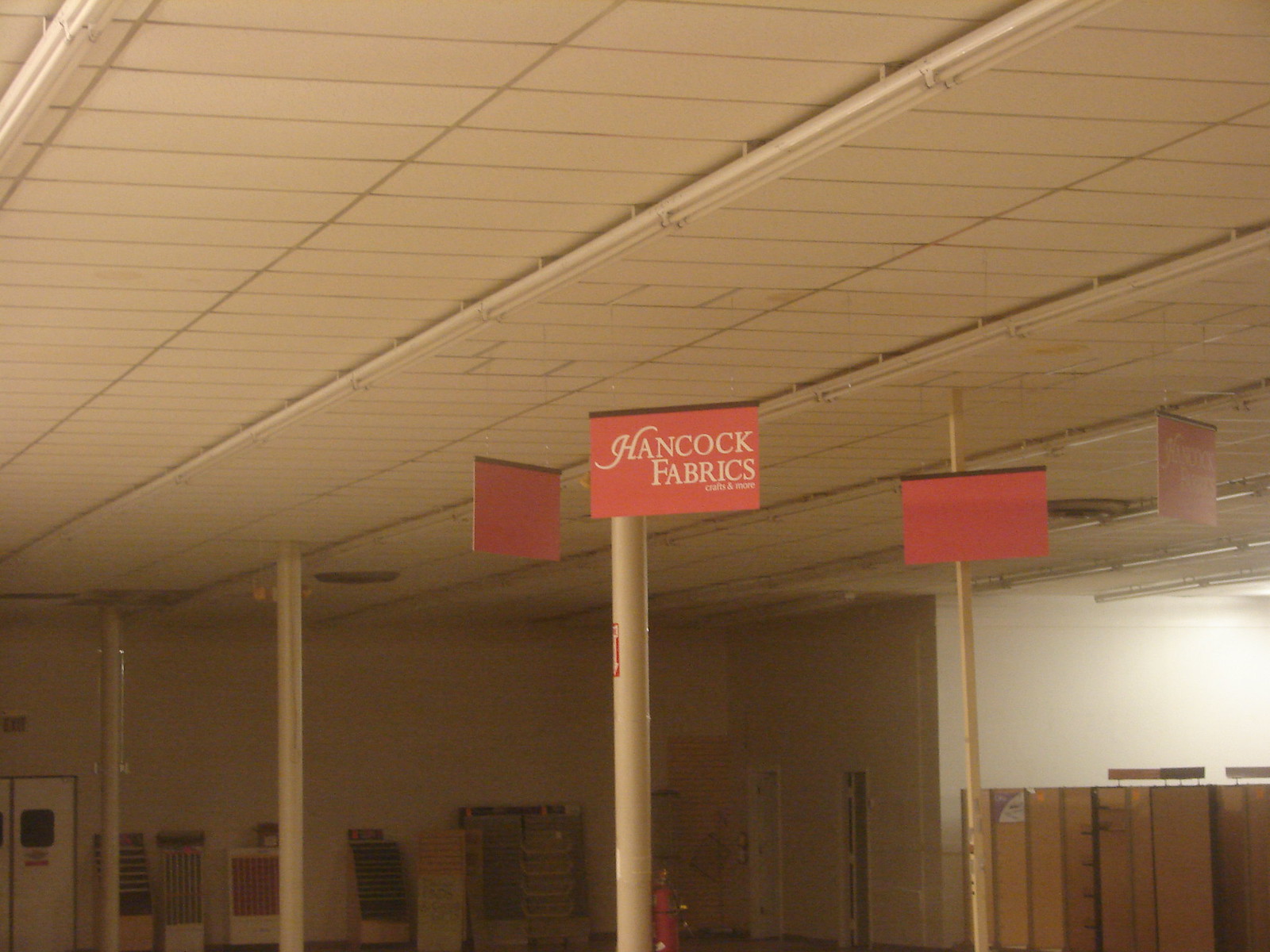This interior image captures a spacious warehouse setting with evident industrial features. Centrally, double doors suggest an entrance into the expansive area, flanked by sturdy metal columns and poles scattered throughout. Overhead, long fluorescent lights illuminate the scene, casting a bright, even glow across the space. Prominent red signs hang from the ceiling, with one clearly displaying “Hancock Fabrics.” To one side, a large window is indirectly visible through its reflection on a nearby wall, though the window itself remains out of the frame. At one end of the warehouse, several boards showcase an array of fabric samples, indicating the textile nature of the business. Cardboard boxes are stacked high near the reflective wall, suggesting ongoing inventory or storage activities. Additionally, a fire extinguisher is mounted on one of the poles, adhering to safety regulations. In the background, other doors lead to different sections of the business, hinting at a larger, interconnected workspace.